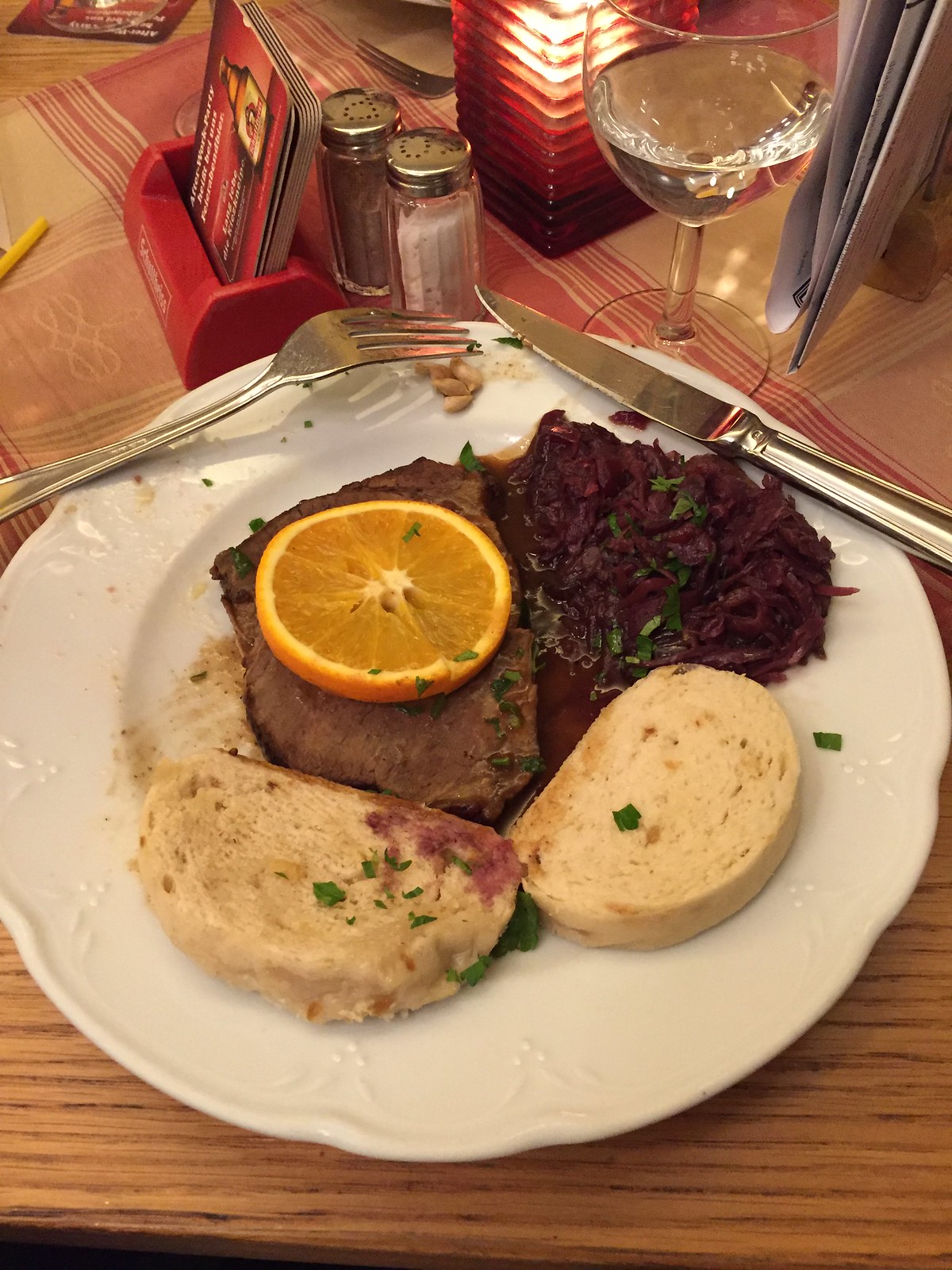The image captures a top-down view of a white circular plate with embossed edges, filled with an artfully arranged meal. At the center of the plate is a cut of beef, topped with a slice of orange. To the right, a reddish-brown or purple heap, likely caramelized onions or red cabbage, adds contrast. Below this, two oval-shaped pieces of bread lie towards the lower portion of the plate. A smattering of green onions or parsley is sprinkled across the dish, adding a fresh, vibrant touch. A fork and knife are neatly positioned at the top of the plate, with the fork on the left and the knife on the right. The plate rests on a wooden tabletop, partially covered by a red and beige striped tablecloth. Above the plate, there is a wine glass filled with a clear liquid, a red tray holding business cards, and a pair of salt and pepper shakers. A small, red decorative candle completes the cozy setting, suggesting a restaurant ambiance.